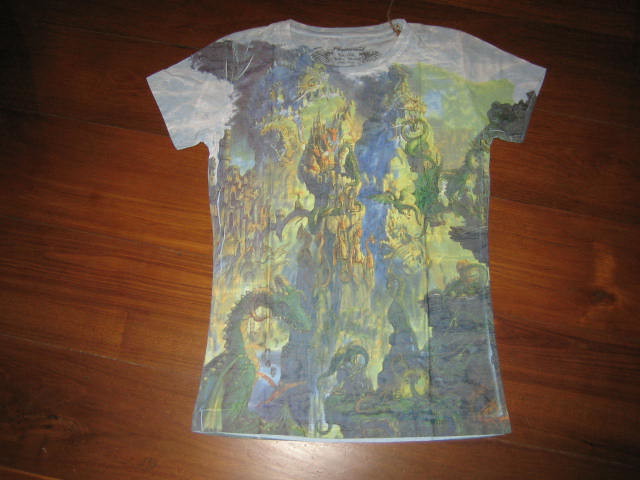This image showcases a neatly laid-out t-shirt on a medium brown floor, which subtly darkens toward the edges of the photograph. The t-shirt is perfectly smoothed out, displaying its elaborate fantasy-themed design in full detail. At the bottom of the shirt, a vibrant green dragon with an elongated neck is depicted, surrounded by jagged rocky crags on the right-hand side. Above this, a grandiose tower emerges, seemingly carved into a massive stone, resembling a fortress integrated into the landscape.

Scattered throughout the scene are numerous green dragons soaring across the fantastical realm. Further in the background, the top left corner of the design hints at a distant icy landmass, possibly an ice shelf, adding depth to the mythical setting. Crowning the image at the very top is a strip of black text, providing additional lore and context to the depicted fantasy world, enhancing the immersive visual narrative.